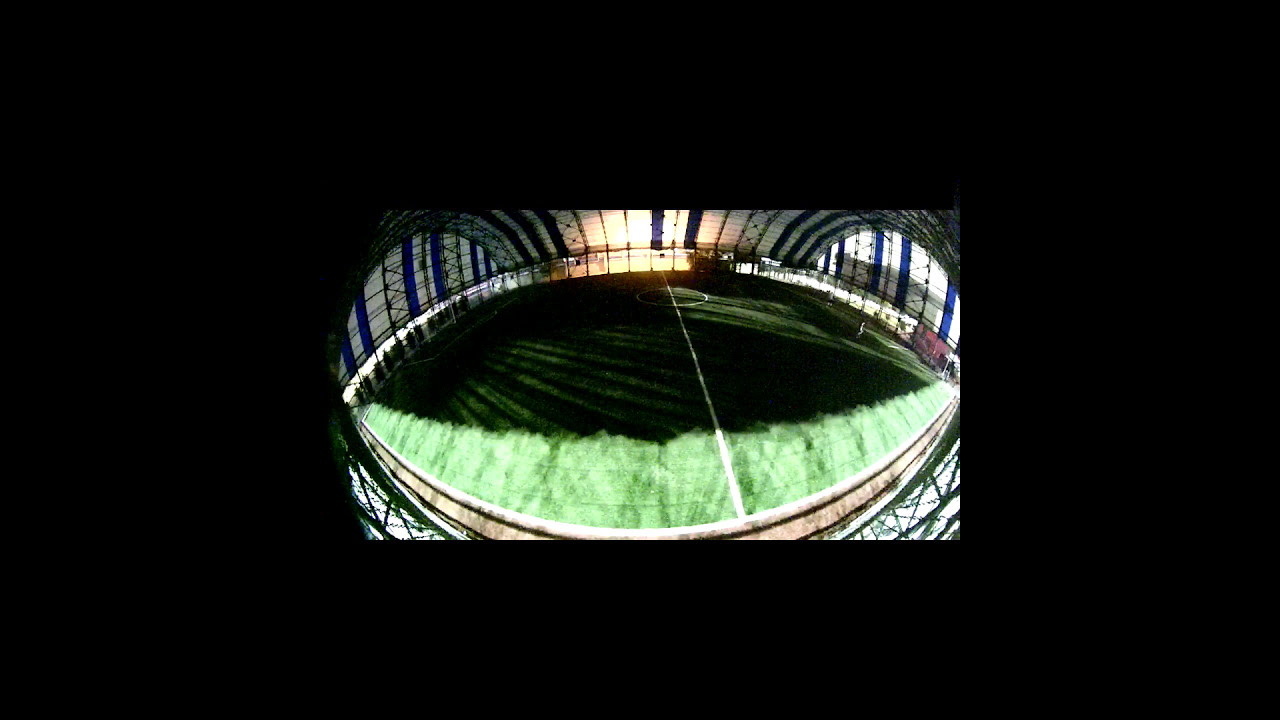The image, taken through a lens, showcases an indoor soccer field, delineated by a prominent black rectangle around the photo's edges, leading to a slightly distorted view. The field itself is lush with green grass and clearly marked with a central white striped midline and a small white circle. The top half of the picture includes blue, black, and yellow stripes that appear to be part of the ceiling or upper structure of the stadium, which is bathed in natural light streaming through the arena windows. A large shadow partially obscures the field, covering nearly two-thirds of it with dark streaks. Additionally, there seem to be faint outlines of figures on the left-hand side, though indistinct.